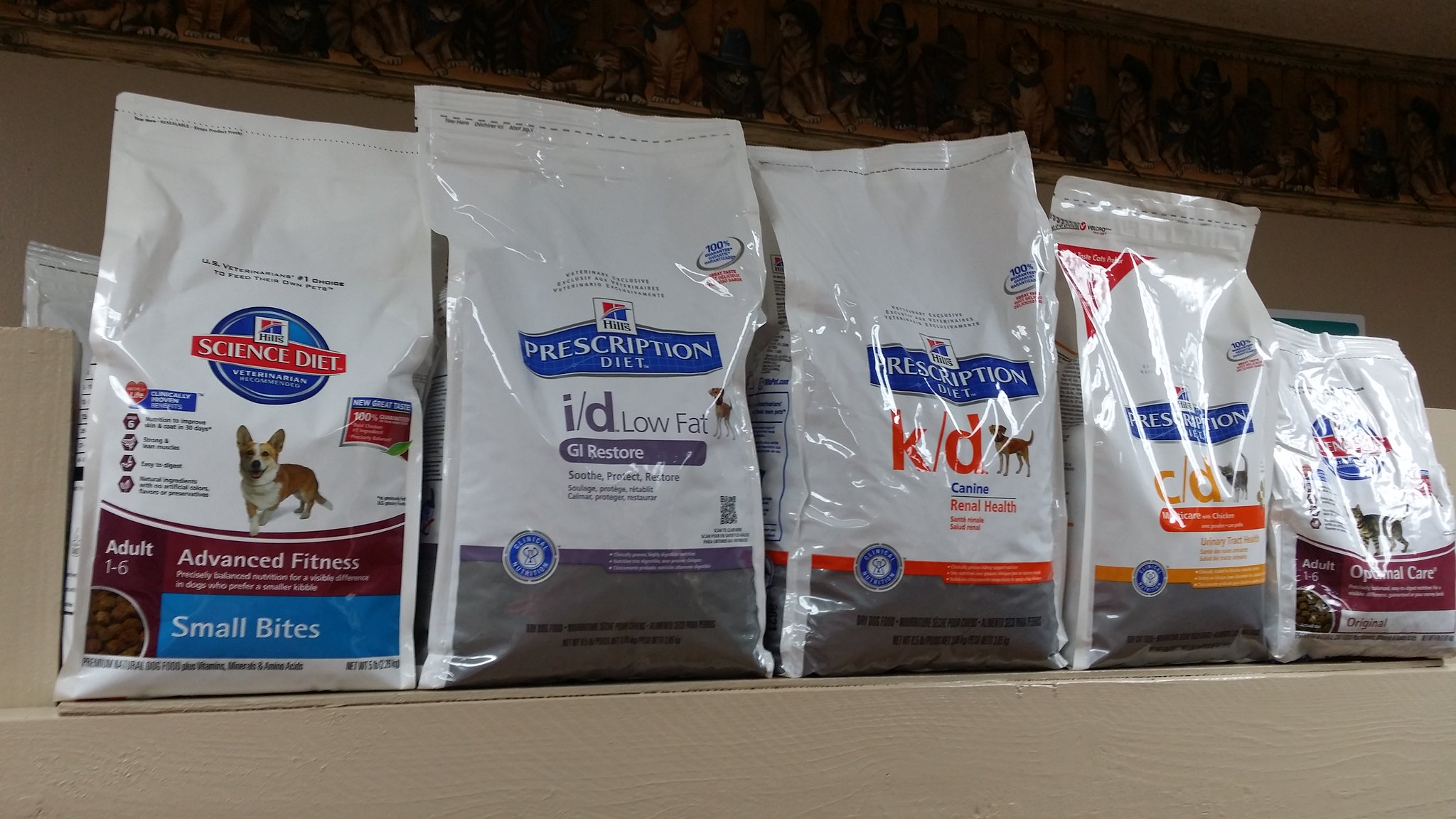The photograph, taken in a low-light room, features five white bags of high-quality dog food meticulously lined up on a beige wooden shelf against a dark brown wall. The first bag stands out with its distinctive design: a blue circle encompassing a "Science Diet" logo in white set on a red background. Beneath this logo, a picture of a corgi dog complements the text "Advanced Fitness Adult 1-6" written in burgundy, purple, and white. Additional details include "Small Bites" in a blue box and a small picture of kibble at the corner.

The second and third bags prominently display the "Prescription Diet" label. The second bag is marked as "ID Low Fat GI Restore" with a gray bottom, and although a dog image is present, it is not clearly identifiable. The third bag, similar in design, is labeled "K-D Renal Health" with the "K-9" marking and features a gray bottom with a red stripe above it.

A glimpse of the fourth bag reveals the "Prescription Diet" label and "C-D" in yellow, accompanied by an unclear dog picture. The final bag, partially visible, also bears the "Prescription Diet" label and the words "Optional Care" at the bottom. Each bag is part of a premium animal food lineup, suggesting a pet store setting where these specialized products are available for sale.